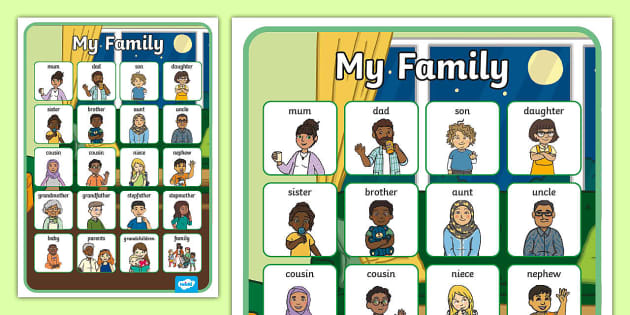The image depicts a cartoon-style family tree, split into two sections displayed side-by-side. At the top of each section, "My Family" is written in white letters against a green background. The background also features a window showing a crescent moon and stars in a blue night sky, framed by yellow curtains.

On the left side, the full family tree is visible. This section includes rows of cartoon characters with labels. The first row features a brown-skinned woman labeled "Mom," wearing a purple jacket over a white shirt. Next to her is a black man labeled "Dad," depicted with a fuzzy beard and wearing a blue jacket over a white shirt. Adjacent are "Son," a yellowish-skinned boy with fuzzy hair making a fist bump, and "Daughter," who resembles Velma from Scooby-Doo with short hair and glasses.

The next row has titles and images for "Sister," "Brother," "Aunt," and "Uncle." Following that, another row includes "Cousin," "Cousin," "Niece," and "Nephew." The right half of the image zooms in on a portion of this family tree, making the images and labels more visible. In addition to the characters, the right section also typically features two more rows listing other family members, which may include "Grandmother" and "Grandfather." This detailed cartoon visualization effectively organizes and labels an extended family structure.